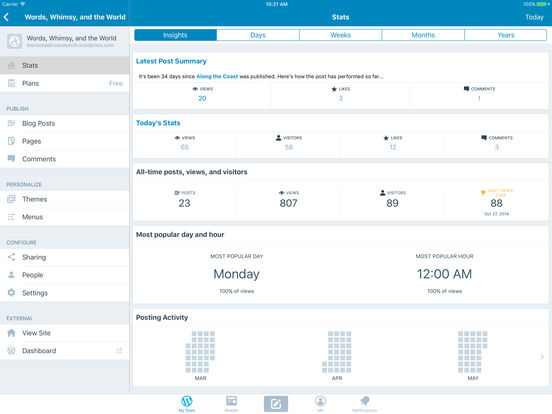The image depicts a computer screen showcasing what appears to be a WordPress dashboard for a blog or website titled "Words, Whimsy, and the World." On the left panel, there are various tabs labeled Stats, Plans, Blog Posts, Pages, Concerns, Thomas, Marius, Sharing People's Settings, View Safe (possibly), View Something (likely), and Dashboard. The central area of the screen displays several sections: Latest Post Summary, Today's Stats, All-Time Post Views and Visitors, Most Popular Day and Hour, and Posting Activity. The distinct WordPress logo suggests this is a content management interface where the site owner monitors the performance and engagement metrics of their blog.